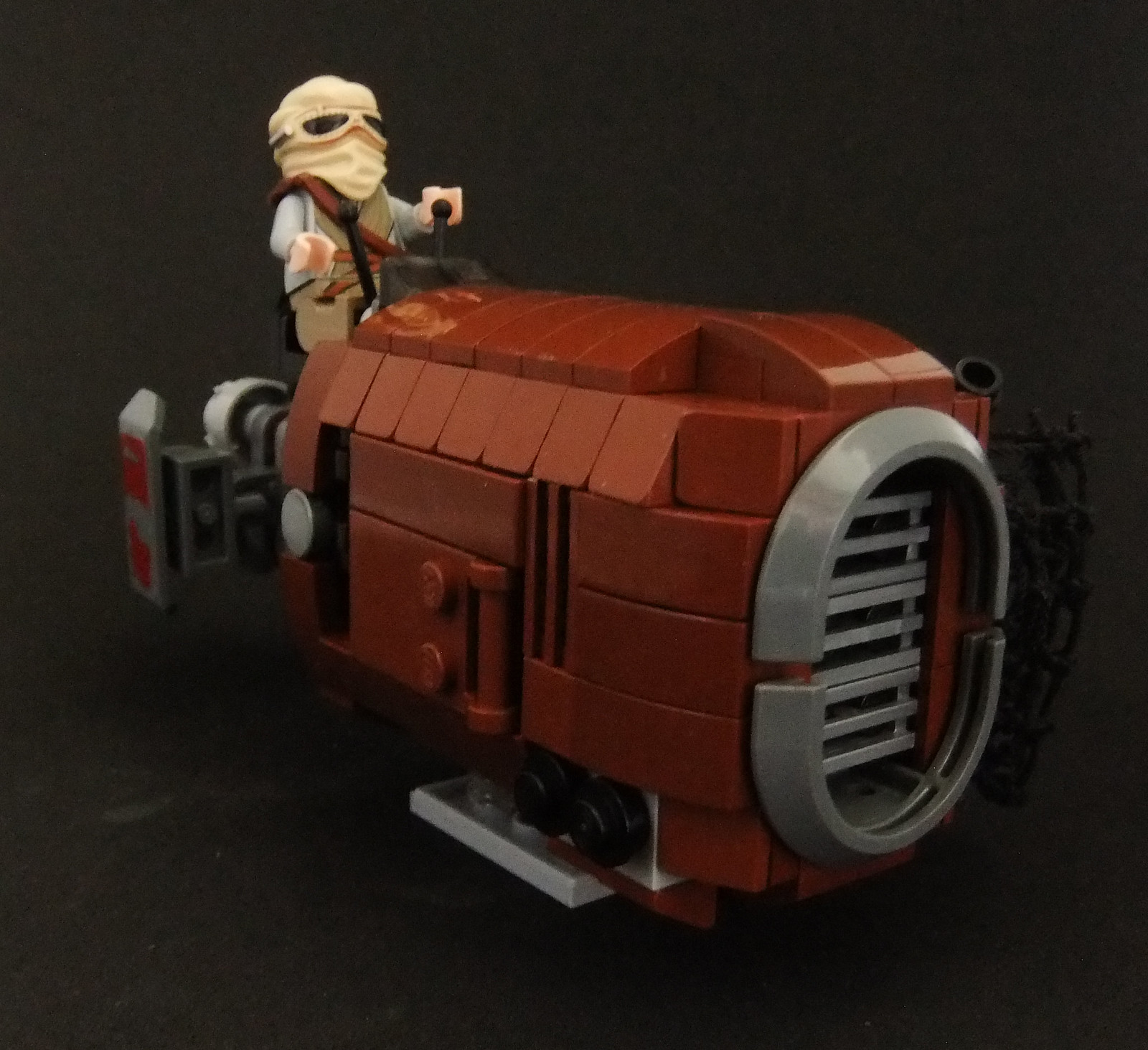This photo depicts a meticulously assembled Lego Star Wars set, featuring a vehicle reminiscent of a speeder from "Return of the Jedi." The speeder has a robust, thicker body with a distinctive design. Its construction includes a brown and orange color scheme with a gray, oval-shaped front that resembles a helicopter's propeller. The speeder is equipped with a silver grill at the front and a prominent jet engine at the back. It sits on a black platform against a dark charcoal gray background, highlighting its details.

Seated in the vehicle is a Lego figure, which adds a touch of character to the set. The figure is dressed in a tan or beige robe and sports a cream-colored cloth mask that covers its face, leaving only the eyes visible through black cutouts. The attire suggests the figure is prepared for a sandy environment, with additional details such as a brown leather-like sash across the torso. The figure's pale hands grasp a pair of black controls, showcasing its role as the pilot of this impressive Lego model. The overall scene is minimalistic yet rich in detail, emphasizing the intricate features of this small but captivating Star Wars-themed Lego set.